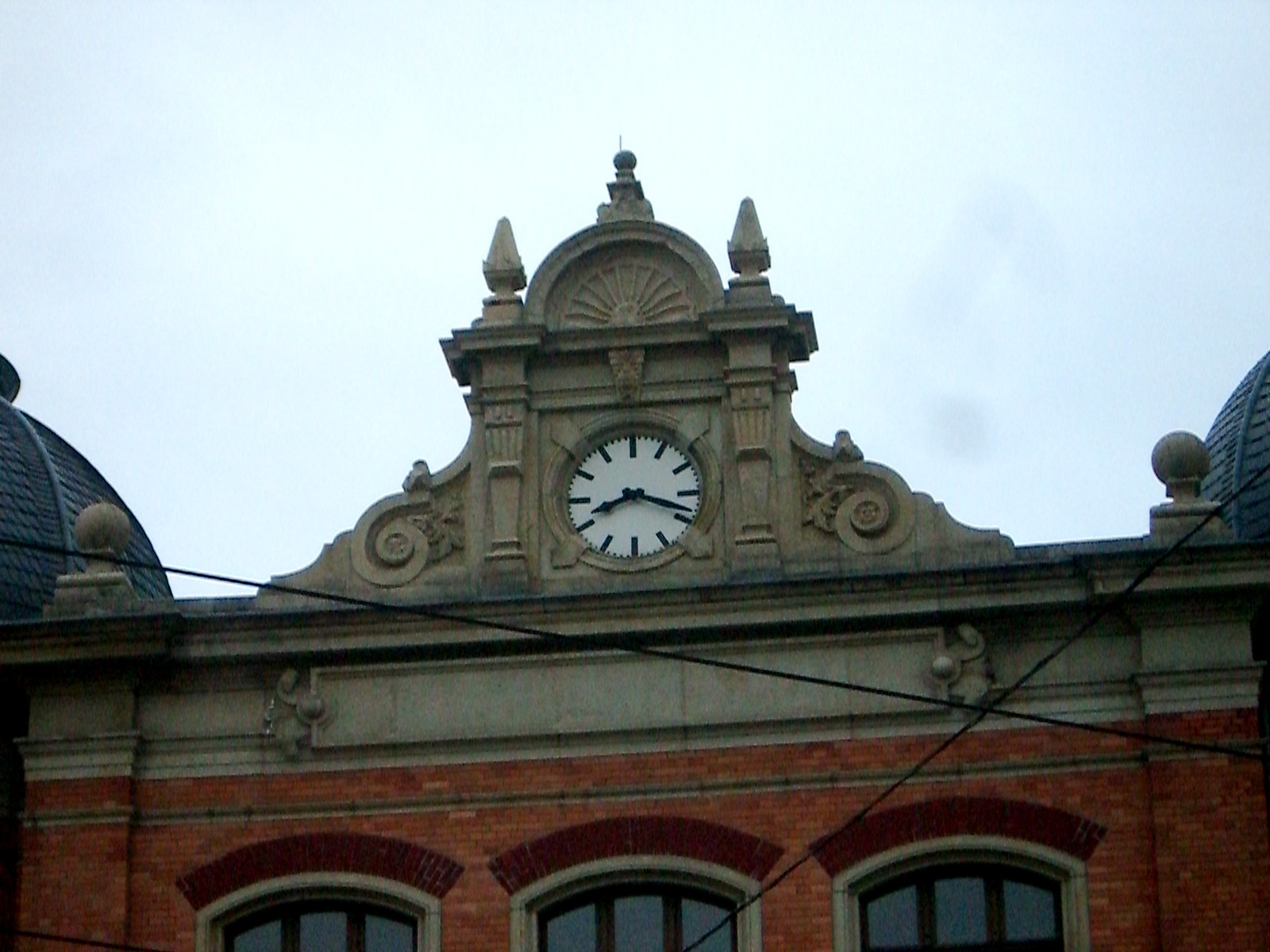This photograph captures the upper portion of an older, ornately designed building constructed with red bricks. The bottom segment of the image reveals the tops of three slightly arched windows, each divided into three individual panes. 

Dominating the center of the image is a grayish stone or concrete structure capping the building, atop which sits a detailed clock tower. The clock boasts a white face with black hands and simple dashed markings to denote hours and minutes. The clock indicates the time as 8:19.

On both the left and right sides of the image, small domed sections of the building are visible, covered with dark grey-blue tiles arranged in a detailed pattern. The backdrop of the photograph features a bleak, light grey sky, suggesting overcast weather conditions and a generally gloomy atmosphere.